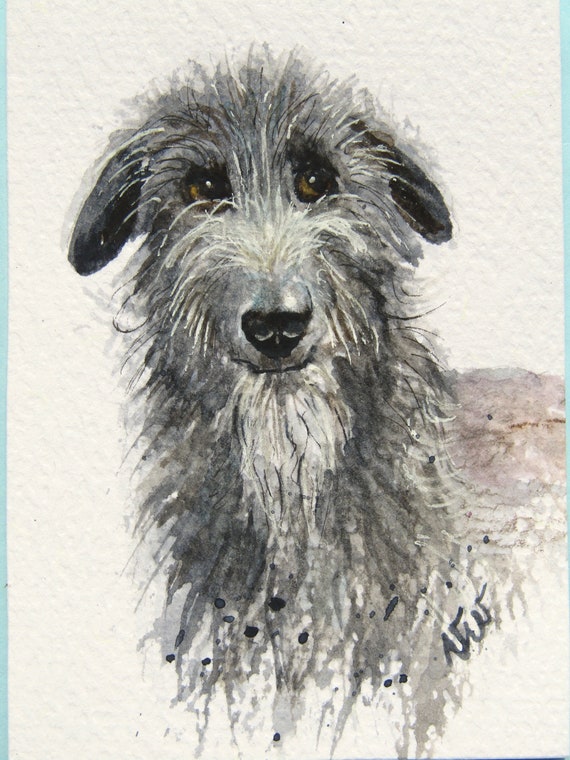The image is a vertically oriented watercolor painting of a small, furry dog, likely from the terrier family. The dog, which has medium-length hair, is depicted from the top of its head down to part of its upper body, fading out into the white background. It features a mainly grey and white coat with patches of pink on the right side of its body, and very dark grey, almost black, ears. The dog's eyes have a golden-yellow tint, and its face, characterized by shaggy hair, gives it an almost bearded appearance with a wider patch of white fur below its mouth and above its nose. The dog is looking directly at the viewer with a direct, neutral expression. The background has the texture of watercolor paper. The artist's initials, which appear to be "VW," are signed in script in the bottom right-hand corner.